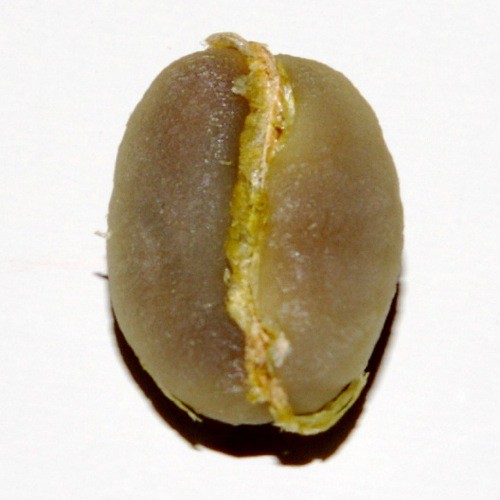The image features a vertically aligned, brown, oval-shaped item with a somewhat transparent, jelly-like exterior. Positioned against a white background with a shadow cast towards the bottom, the item bears a striking resemblance to a hamburger bun at first glance. However, it more closely resembles a type of food that seems unfamiliar. This item is characterized by a central, goldish-yellow, creamy stripe that starts near the left side, curves down the middle, and veers towards the right, possibly indicating an egg-like filling or root wrapping around it. The central stripe appears integrated with the piece, suggesting it may have formed or emerged during cooking. Additionally, there is a small, black portion protruding slightly from underneath the item, adding to its unique appearance.